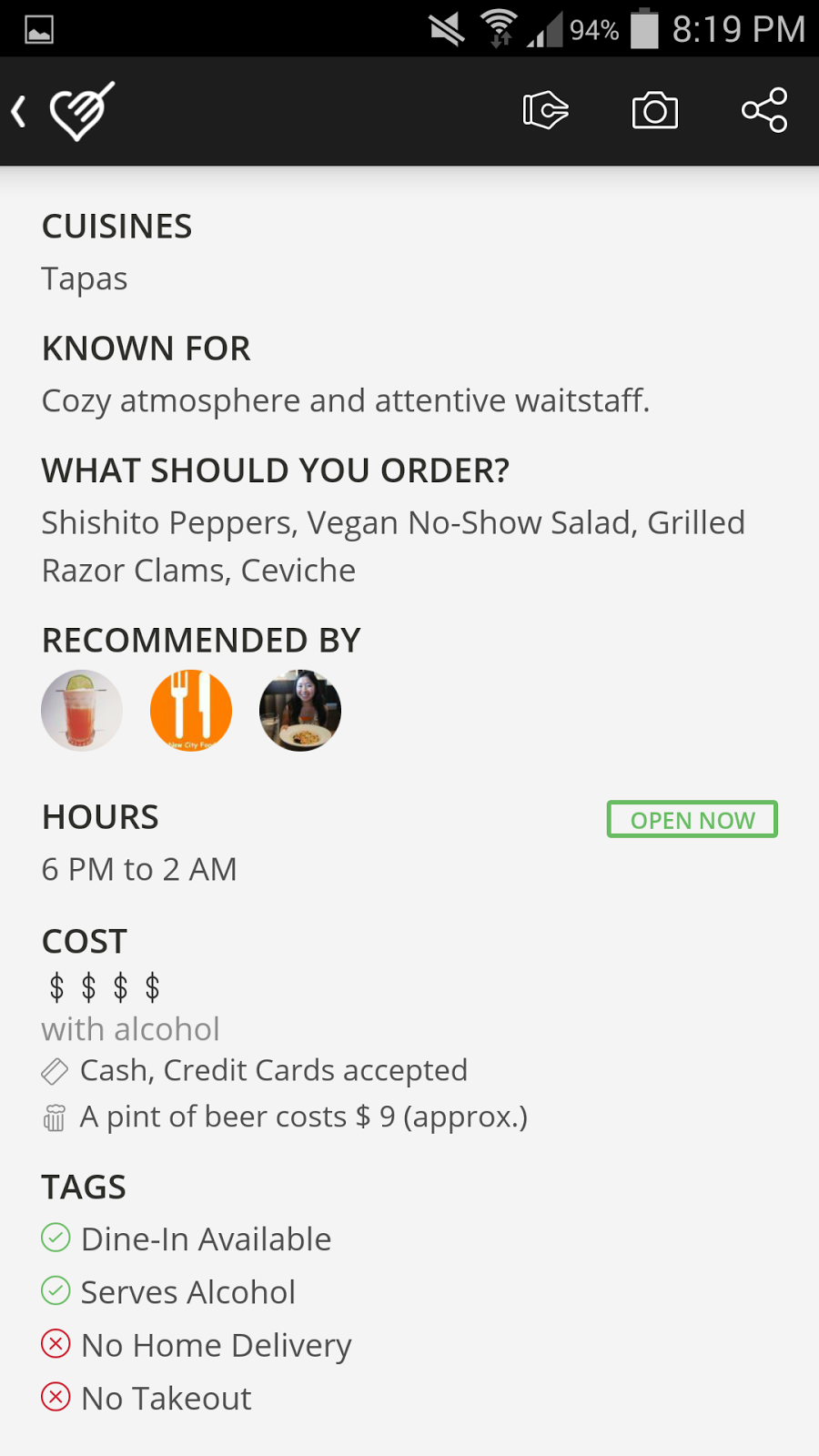This is a detailed caption for a cell phone screenshot taken at 8:19 PM, showcasing a restaurant's overview and details. 

At the top of the screenshot, there is a black rectangle featuring white icons and light gray text. Below this, on a light gray background with black font, the word "Cuisines" is displayed in all caps. Underneath, in a slightly lighter font, it reads "Tapas".

Further down, in all caps black font, it states "KNOWN FOR," followed by slightly smaller gray font that reads, "Cozy Atmosphere, [in] a Tin of White Stuff". 

Next, in all caps black font is the prompt, "WHAT SHOULD YOU ORDER?" Below this, written in gray, slightly smaller font, are dish recommendations: "Shishito Peppers," "Vegan No-Show Salad," and "Grilled Razor Clam Ceviche."

Following this, the text "RECOMMENDED BY" appears in all caps black font, accompanied by three user avatars represented as circles. To the right, there is a green-outlined rectangle with all cap green font indicating "OPEN NOW."

Underneath is a section labeled "HOURS" in all caps black font, followed by smaller gray text specifying the hours of operation: "6 PM to 2 AM." Further down, in black all caps, it reads "COST," with four dollar signs beneath it signaling a high price range. Below this, it mentions "with alcohol," notes that "Cash and Credit Cards Accepted," and mentions a pint of beer costs approximately nine dollars.

Lastly, the section "TAGS" is in all caps black font, followed by green-checked options "Dine-In Available" and "Serves Alcohol." Additionally, "No Home Delivery" and "No Takeout" are marked with an X.